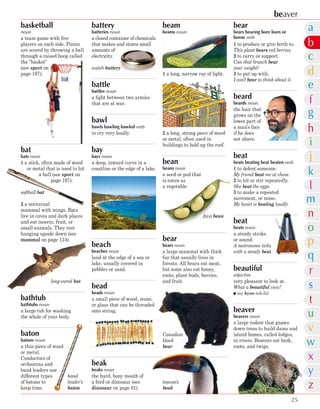This detailed image from a textbook page showcases an alphabetized list of terms with corresponding pictures, primarily related to various structures, people, sports, animals, and musical instruments. On the top left, there's an illustration of a basketball player about to dunk a ball, labeled "basketball." Nearby, on the top right, it says "beaver" with a red line beneath it, and a picture of a beaver is shown. Just below this, a black bear facing left is depicted with the word "bear" adjacent to it. In the center top, a small cell battery is shown labeled "battery." Moving right, there's a depiction of a light beam labeled "beam," and adjacent is a diagram of a house’s rafters, also labeled "beam." Left of the beam, labeled "Patrick," is an image of a man who presumably resembles or is named Patrick. Below the center, a diagram of a bird used in sports and animal logos can be found, with the term "bird" accompanying the images. Further down, the image contains colorful representations of 'ball', 'bat', 'bay' with blue crystal water, 'bean' pod with white beans, 'baton' with gold edges, beads, a toucan, and a metronome. Detailed terms such as "beak," "basketball," "button," "battle," "beard," "beach," "bathtub," and "beautiful" are also present, each matched with vivid pictures to aid understanding. This intricate layout of images and text exemplifies how the dictionary page elucidates multiple meanings and representations for each term. The colors used in the text—black, brown, green, yellow, and orange—enhance the visual appeal and clarity.